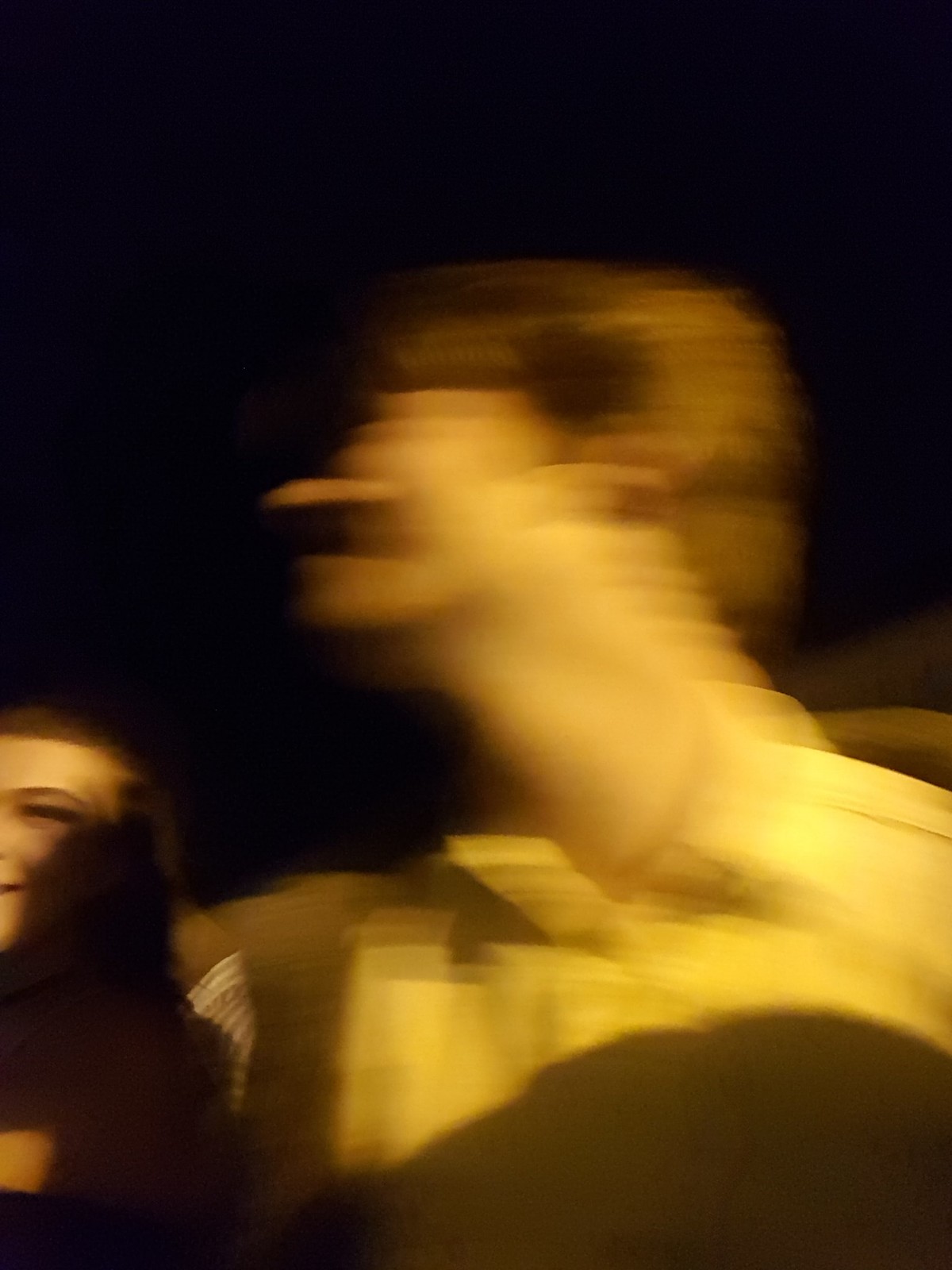An out-of-focus side profile of a man dominates the image, making it difficult to discern his features. He appears to be wearing a white and black button-up shirt with a V-neck and turtleneck beneath, but the details are obscured. To his left, a more distinguishable, clear-faced woman looks towards the camera with a slight smile. Her facial expression is directed forward, partially turned towards the photographer. Her attire remains indiscernible due to the framing. The man's blurred visage gives an illusion of a mustache, adding to the overall ambiguity of his appearance.